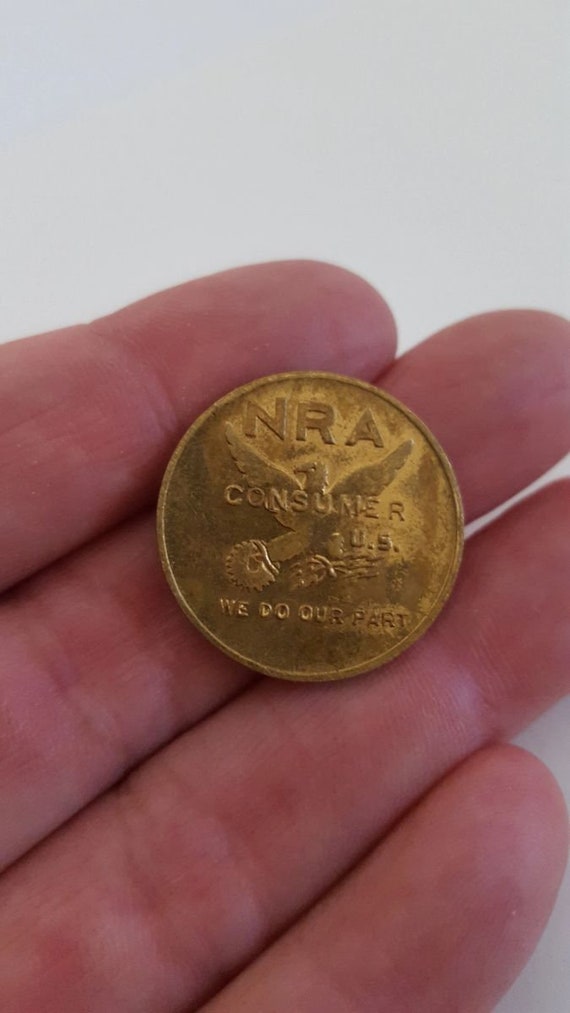The image is a detailed digital photograph depicting a close-up of a partial hand, specifically four fingers of a Caucasian person, emerging from the left-hand side and extending toward the top right. The background is mostly a white or off-colored blue, giving a slightly tarnished or aged appearance, while the focus is on the hand palm-upholding a large, yellowish gold coin. 

The coin is positioned across the middle and ring fingers, with text inscriptions and an emblem on it. At the top of the coin, the initials "NRA" are prominently displayed. In the center, the word "Consumer" is inscribed, with the letters "US" directly below. Toward the bottom of the coin, the phrase "We do our part" is clearly visible. 

Notably, the coin features an emblem of a bird, likely a dove or an eagle, positioned behind the text. The bird appears to be looking to the left, and though partially obscured by the text, it holds two indistinct objects in its talons. The overall texture and color of the coin suggest that it might be old and tarnished.